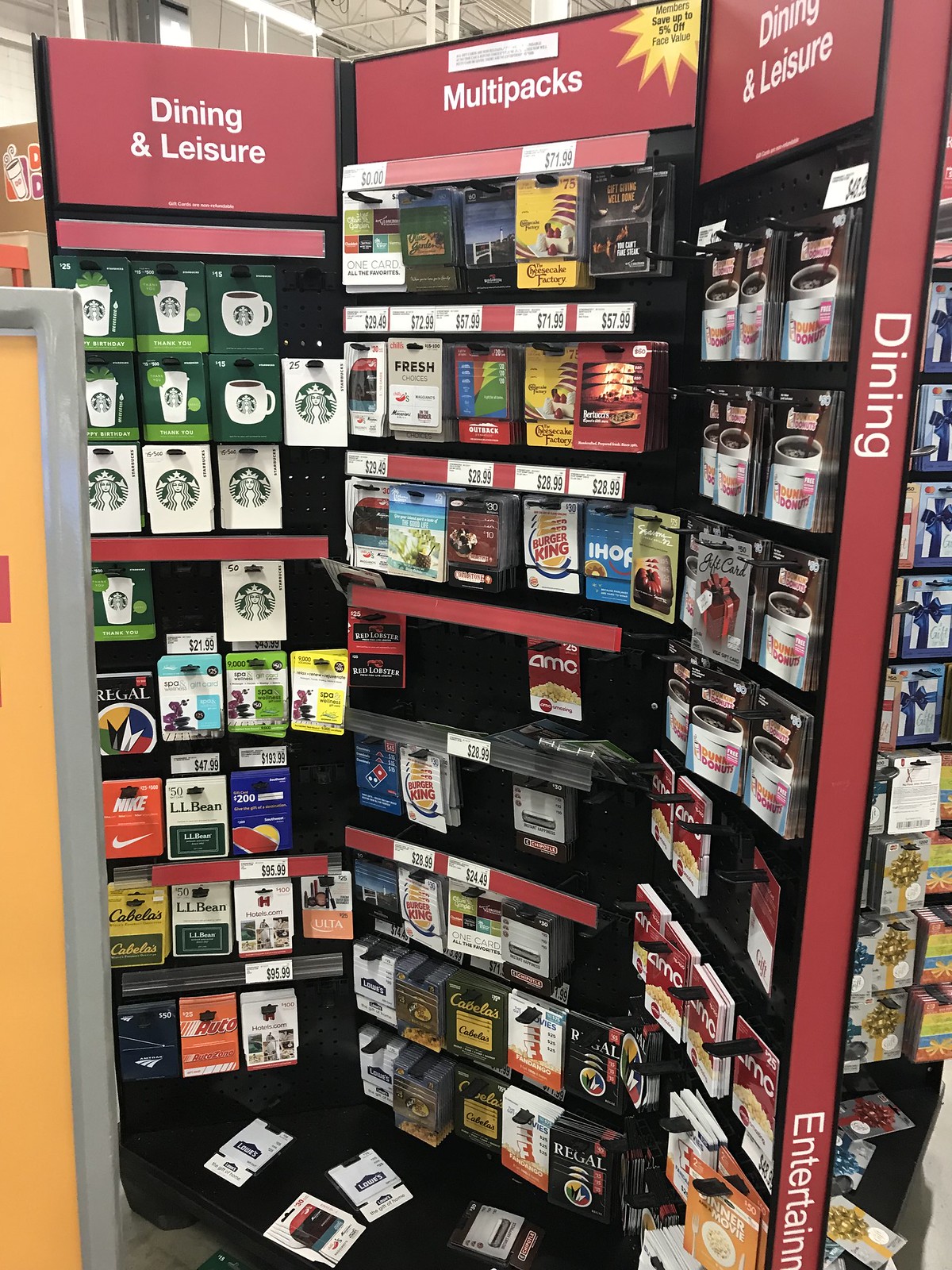The image showcases a rotating gift card display commonly found in grocery and retail stores. The display's frame is vibrant red, and it features three distinct sections, each encased in red-bordered boxes. To the left, the section labeled "Dining and Leisure" exhibits an array of Starbucks gift cards, distinguished by their iconic green and white backgrounds. Below these, additional gift cards related to dining and leisure are visible, complete with price tags. The central section, marked "Multipax," presents a variety of branded gift card packs from well-known businesses such as IHOP, Burger King, Domino's, and AMC. Notably, this section includes a promotional message inside a yellow sun-like design that reads, "Members save up to 5% off face value." The right section, also labeled "Dining and Leisure," predominantly showcases Dunkin' Donuts gift cards alongside AMC movie theater cards.